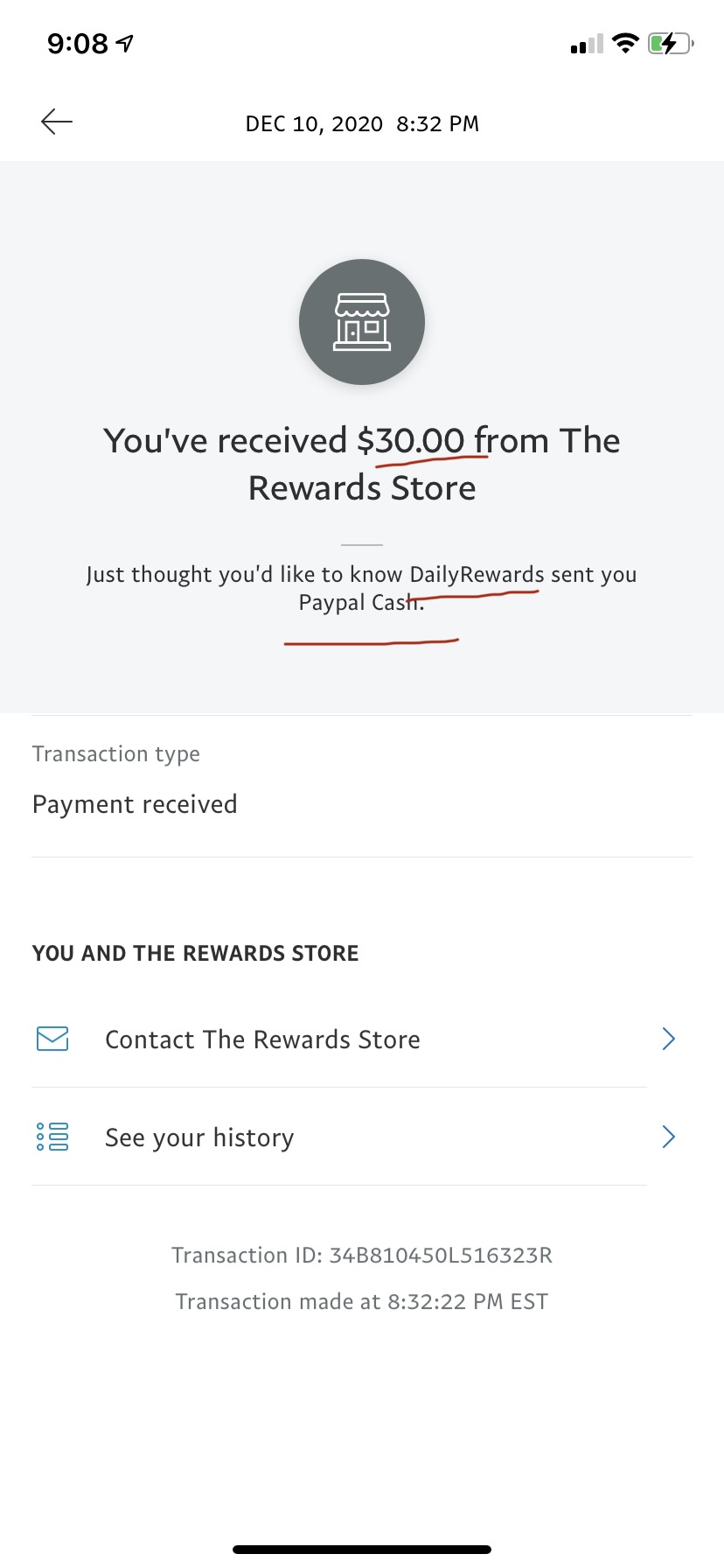The image depicts a digital interface, possibly a screenshot from a rewards or survey site. The top section of the interface displays the current time, 9:08, a lightning bolt indicating that the device is charging, and Wi-Fi connectivity status. 

Below this, a transaction history is shown, specifically highlighting an entry on December 10th at 8:32 PM. There's a prominent gray box with the message: "You received $30 from the reward store," accompanied by smaller text that states, "Just thought you’d like to know the daily rewards that you pay for cash." Additionally, key phrases “$30,” “daily rewards,” and “PayPal cash” are underlined in red, likely hand-drawn for emphasis.

Further down, the interface provides details on the transaction type, stating "Payment Received" in gray text. In bold, all-caps text, it declares, "YOU HAVE THE REWARD STORE," followed by an icon of a mail envelope labeled "Contact the Reward Store," with a right arrow indicating it's clickable. Adjacent to this is another option labeled "See Your History," also featuring a right arrow for navigation.

At the bottom, there’s a transaction ID composed of a mix of about 12 characters and a timestamp confirming the transaction occurred at 8:32 Eastern Time. The entire interface is set against a white background, and an arrow is positioned to the left of the December date, allowing users to navigate back.